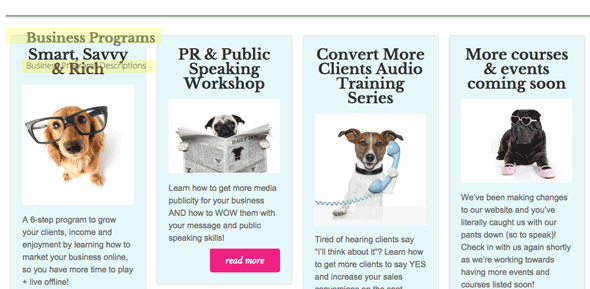The image depicts a page dedicated to business marketing, organized into four distinct sections from left to right. Each section is represented by a light blue rectangle containing a photo, a headline, and text that elaborates on the headline.

1. **Business Program: Smart, Savvy, and Rich**
   - **Photo:** A Golden Retriever or Spaniel type dog wearing oversized eyeglasses, gazing up at the camera.
   - **Description:** "A six-step program to enhance your client's income and enjoyment by teaching you how to market your business online, allowing more time for offline play and living."

2. **PR and Public Speaking Workshop**
   - **Photo:** A pug reading a newspaper.
   - **Description:** "Learn how to secure more media publicity for your business and master the art of public speaking to captivate your audience. An option to read more is available."

3. **Convert More Clients: Audio Training Series**
   - **Photo:** A Terrier type dog holding an old-style phone receiver in its paw.
   - **Description:** "Discover strategies to transform 'I'll think about it' into a 'Yes!' Enhance your client conversion rate and boost your sales. The rest of the description is cut off."

4. **More Courses and Events Coming Soon**
   - **Photo:** A dark-colored Shar-Pei wearing heart-shaped sunglasses and blue shoes on its front paws.
   - **Description:** "We've been updating our website; you've literally caught us mid-update. Check back soon for more upcoming events and courses."